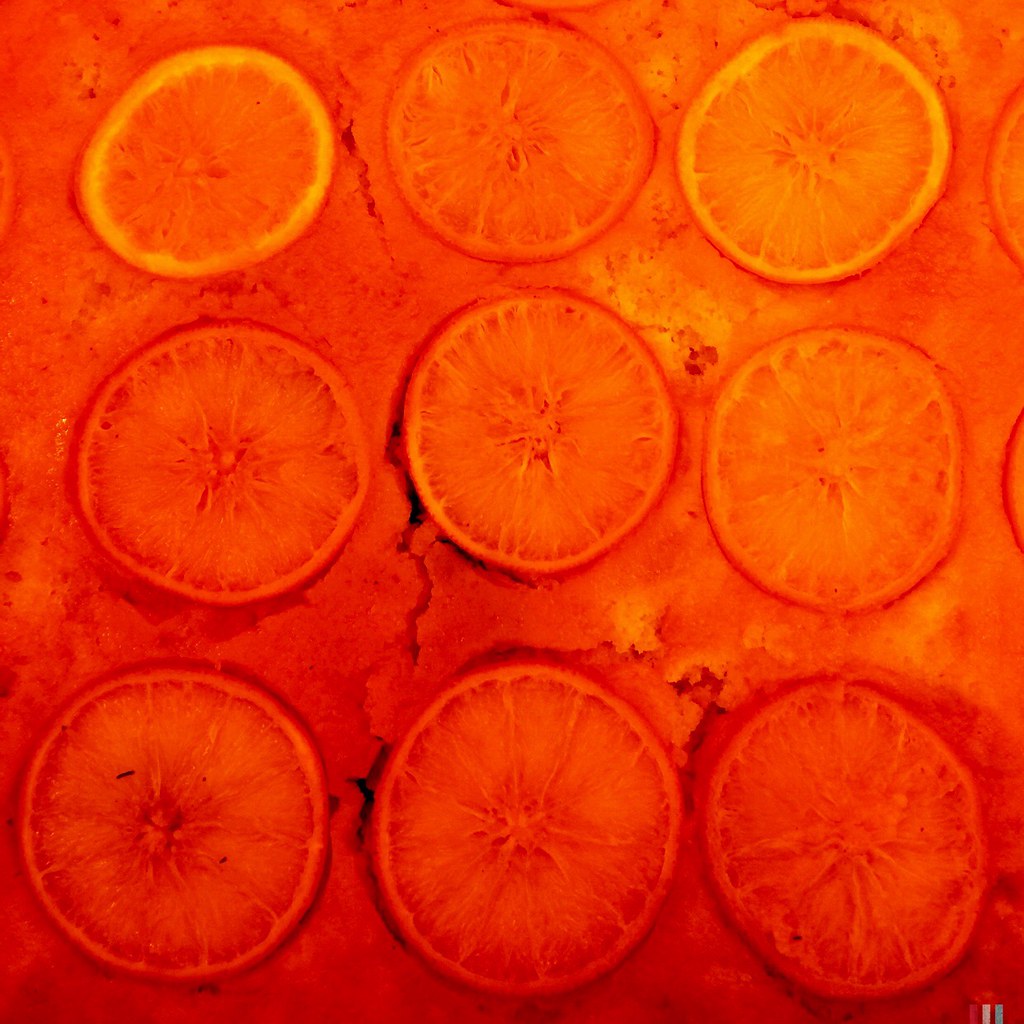This image depicts nine orange halves arranged in a meticulous three-by-three grid, their vibrant interiors facing the camera. Their vivid orange flesh is dotted with visible segments and occasional seeds, revealing the natural texture of each fruit. The oranges rest on a distinctive, rough-textured surface, possibly resembling cracked stone or ice, heavily tinted an intense shade of orange. This background, coupled with overexposed lighting, creates a surreal, almost artistic appearance, with the top-left and top-right oranges appearing lighter and possibly thinner than the others, which contrast with a deeper, richer orange hue. Black spots sporadically grace the background and one of the oranges, further adding to the image's unique and experimental nature.